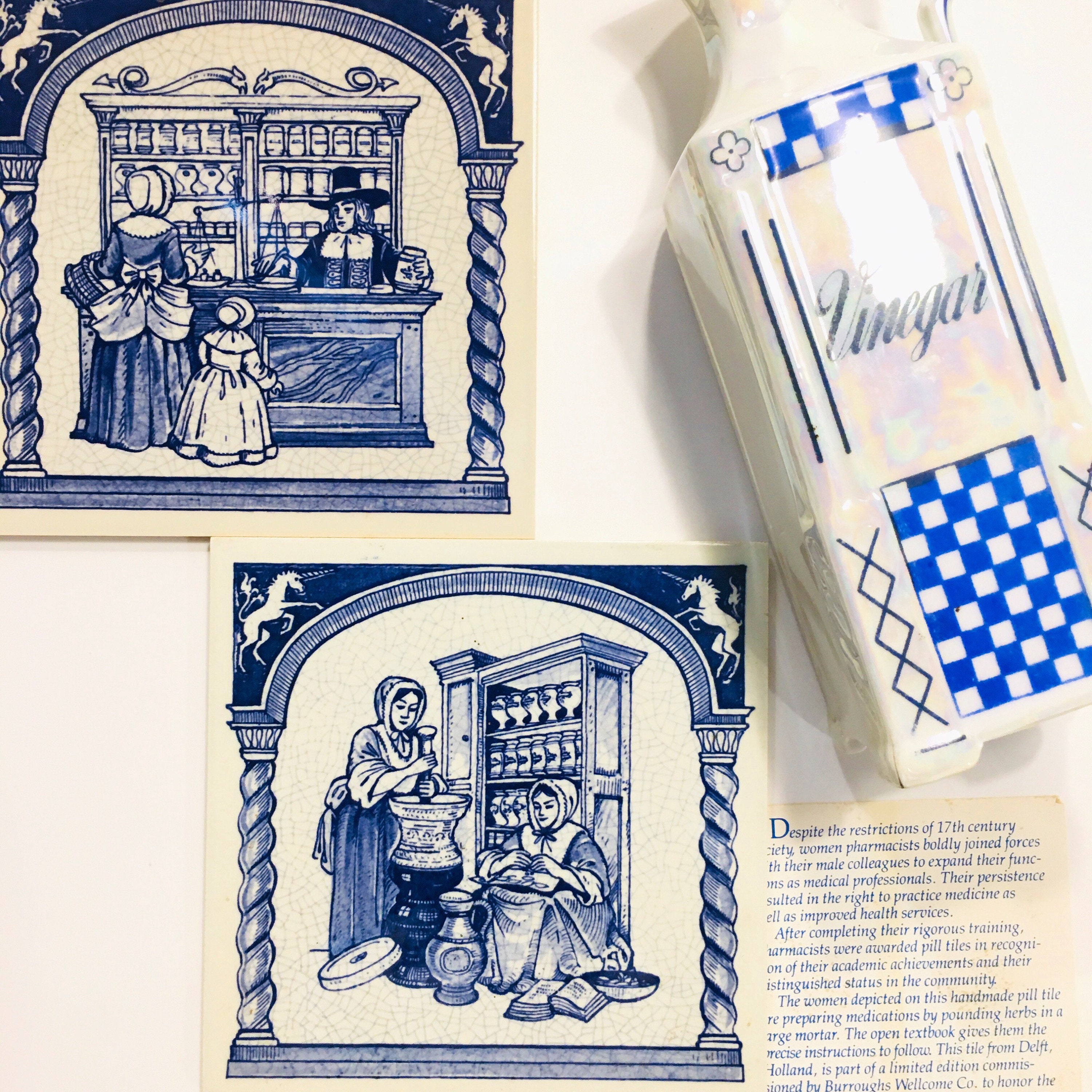This photograph captures a detailed museum exhibition display. Dominating the top right is an antique white ceramic vinegar bottle adorned with a blue and white checkerboard label, suggesting it is a historical artifact. To the left, there are two ornate tiles featuring elaborate dark blue illustrations on a white background. The top tile depicts an early 1700s general store scene with a pilgrim-like shopkeeper assisting a bonnet-wearing woman and her child as they measure goods. An archway and two horses are depicted in the corners, along with two columns framing the scene. The bottom tile similarly features two women; one is using a large mortar and pestle, likely grinding grain, while the other is seated, perhaps preparing green beans by removing the ends and strings. Both tiles are surrounded by an oval crest that mirrors the historical theme. Below the vinegar bottle lies a small informational card, presumably describing the exhibits, though its text is too small to decipher. This arrangement emphasizes the everyday lives and roles of women in historical contexts, possibly highlighting women pharmacists or workers in domestic settings.